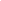This image is completely blank, devoid of any objects, text, or discernible features. Despite thorough inspection, no visible elements can be detected.